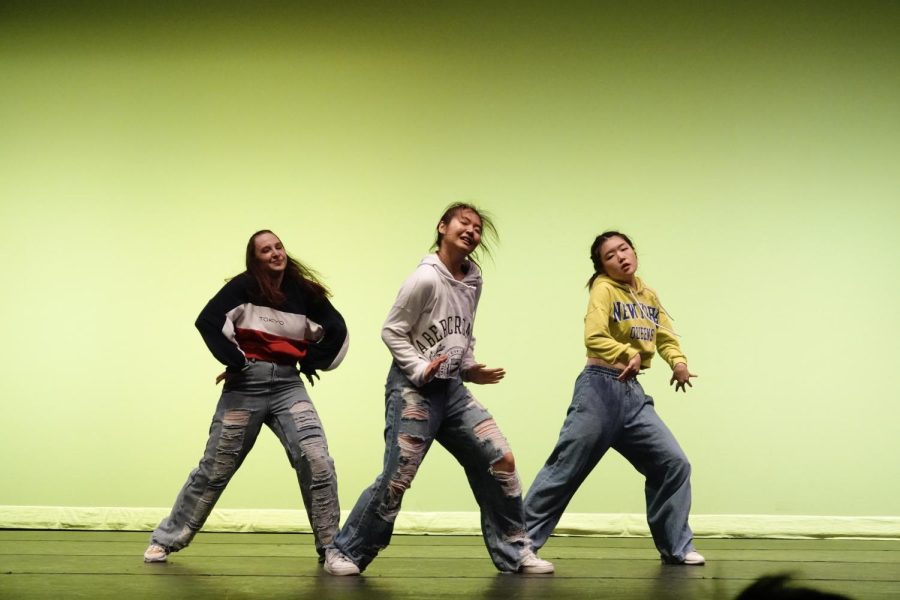In the image, three young girls are dancing on what appears to be a hardwood floor stage, performing a choreographed hip-hop routine. The background features a white and green gradient, along with gray and brown hues. The girls, two of whom are of Asian descent and one Caucasian, all sport streetwear outfits and white sneakers. The girl on the left has long, brown hair down and is dressed in a black, white, and red striped long-sleeve shirt that possibly says "Toronto," paired with ripped long jeans. The middle girl has her black hair tied up, is smiling, and is dressed in a white Abercrombie hoodie with ripped jeans. The girl on the right is wearing a yellow hoodie with "New York" on it, along with gray sweatpants. All three are looking at the camera, striking a pose in their dance routine.